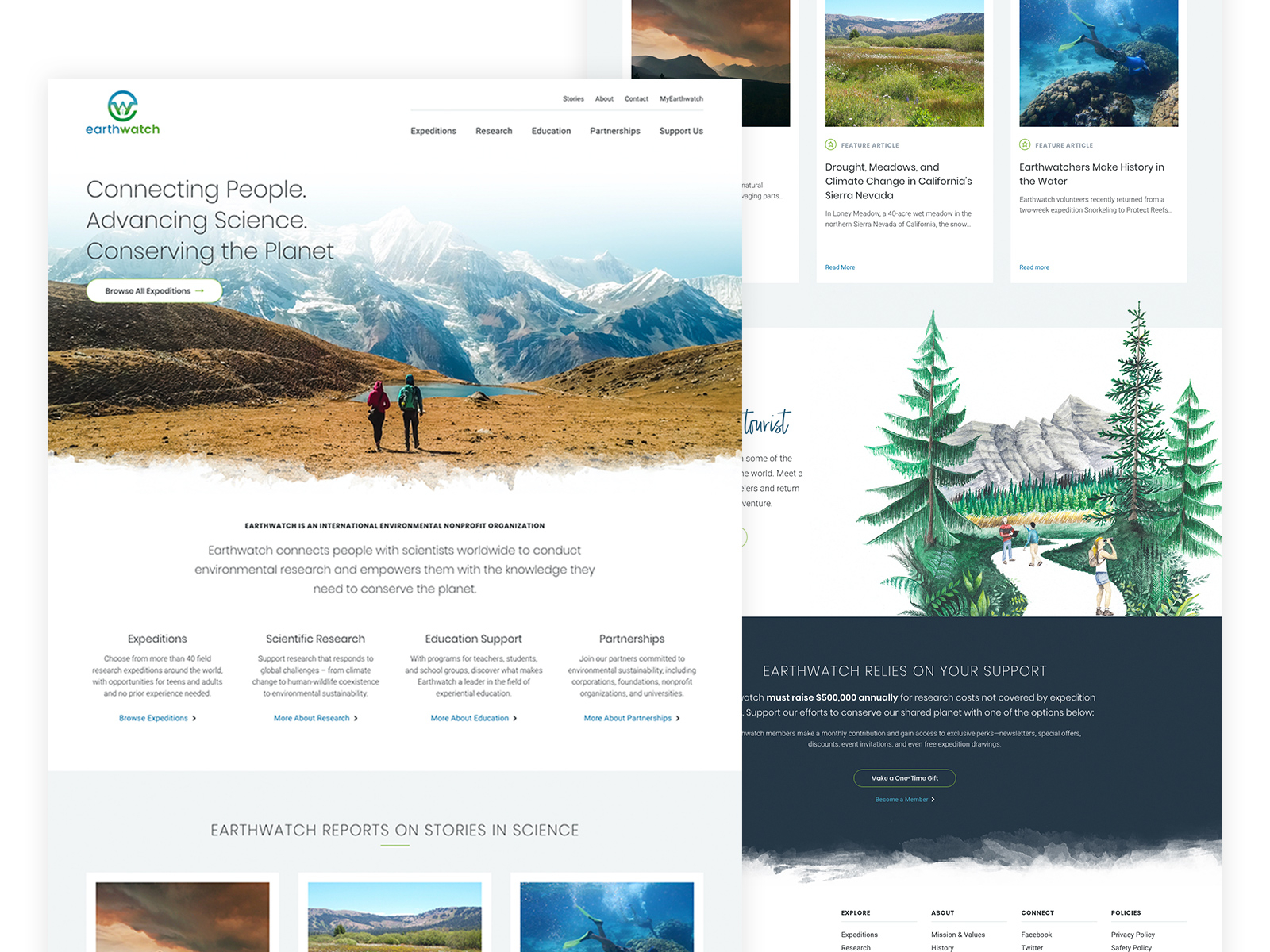This website image features promotional material for Earthwatch, prominently showcasing two slightly overlapping flyers. The flyer on the left is positioned just in front of the one on the right. It includes a vivid photograph of a lush, green landscape with majestic black mountains in the background, a serene small lake, and two individuals walking towards it. The text on this flyer reads, "Connecting People, Advancing Science, and Conserving the Planet." Below this message, a button labeled "Browse All Expeditions" invites viewers to explore further.

At the top right section of the page, there is a navigation menu with the titles: Expeditions, Research, Education, Partnerships, and Support Us. Directly beneath this menu, four distinct sections provide additional information on various Earthwatch initiatives, including expeditions, scientific research, educational support, and partnerships.

Towards the bottom of the page, a section titled "Earthwatch Reports on Stories in Science" displays three partial images, each presumably linked to articles or stories about recent scientific findings. The flyer on the right mirrors these three images but includes short descriptions and titles for each of the stories, although only the second and third images are visible due to the left flyer overlapping the first image.

At the very bottom of the page, there is a statement emphasizing the organization's dependency on public support: "Earthwatch Relies on Your Support."